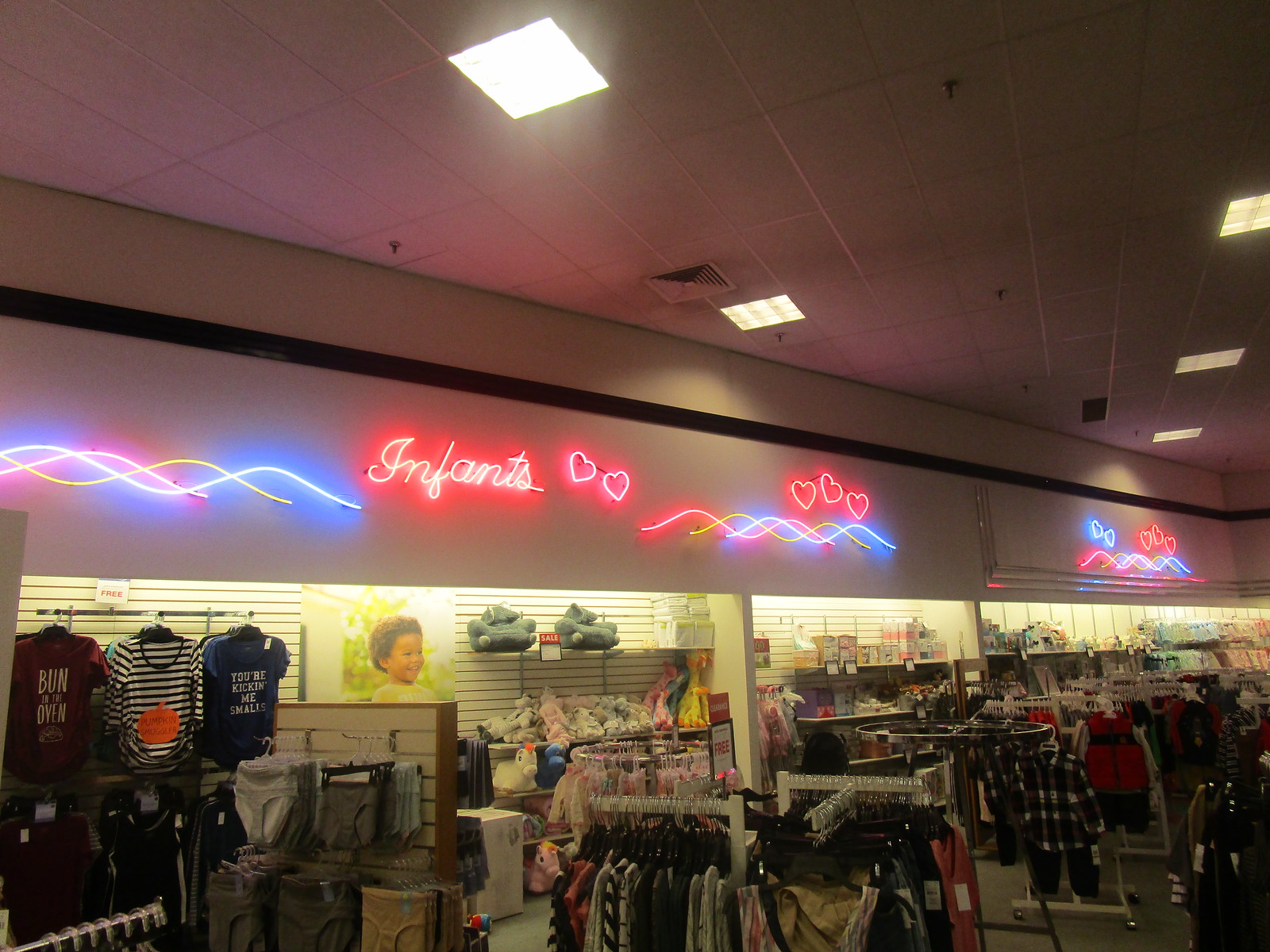The image captures the infants section of a dimly lit clothing store. Prominently displayed on the top part of the wall is a neon LED sign that reads "infants," surrounded by decorative elements such as hearts in red and blue, and wave-like lines in red, yellow, and blue. The overall atmosphere appears to be taken in the evening or just before the store is fully lit. The store has white walls and a white tile ceiling with a scattering of lights shining through. 

In the background, a large picture of an African American infant wearing a yellow shirt and smiling outdoors adds a welcoming touch. The store features various racks filled with diverse infant clothing in colors like red, black, white, pink, and green. Beneath the neon signage, some racks are wall-mounted while others stand freely in the center of the store. Shelves also display an assortment of clothes, and there are a few stuffed animals along the back wall, adding to the playful and engaging ambiance of the infants section.